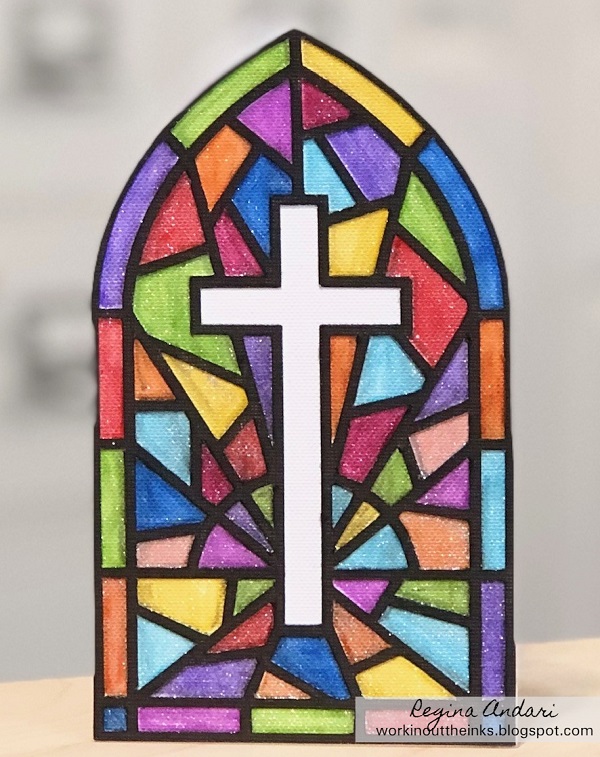This image features a richly detailed, multi-colored stained glass window resembling those found in churches. The window takes the shape of a pointed arch, which rounds out before ending in a straight vertical drop, similar to a door or tall window. The vibrant palette includes shades of blue—both light and dark—orange, pink, red, yellow, green, peach, and purple, set in a dark metal framing typical of stained glass designs. At its center is a white religious cross with a black outline, through which the background, blurred and gray, is visible. The artwork rests on a light-colored beige countertop. In the bottom right corner, the cursive watermark reads "Regina Andari, workingouttheinks.blogspot.com."